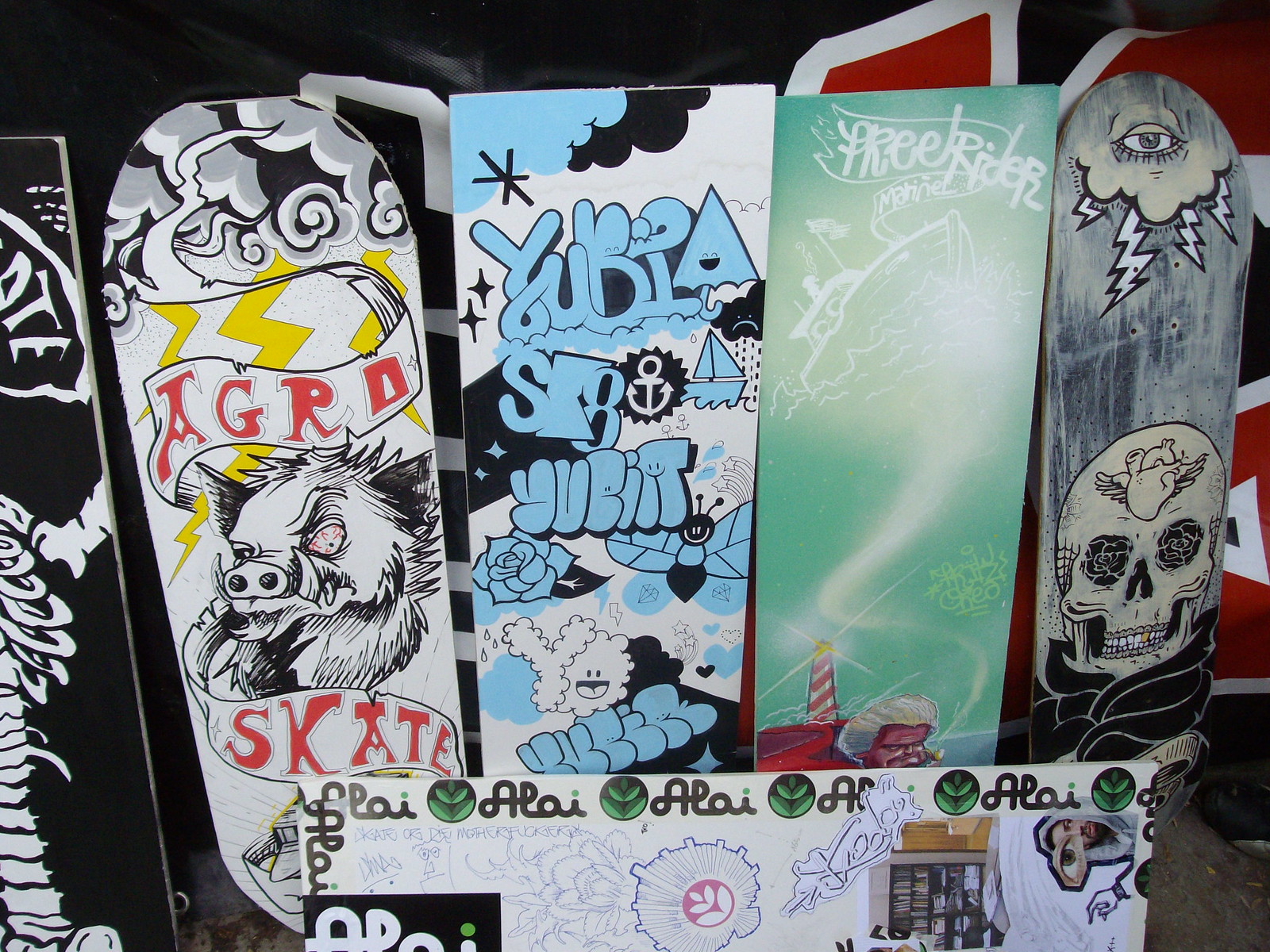The image showcases an eclectic collection of six boards leaning against a black wall adorned with white and red graffiti. Five of the boards are detailed with vibrant urban graffiti art, each exhibiting unique artwork and colors. The first board, partially out of frame, is black with a white scorpion-like figure. The second board, which is slightly rounded at the edges, prominently features a black and white background with red text "Agro Skate" and an illustration of an animal with tusks, along with yellow lightning bolts. The third board, mostly white, displays blue and black graffiti-style writing. The fourth board, light green, depicts a red and white lighthouse with an adjacent large head and an illuminated sky. The fifth board presents a skull and crossbones beneath lightning emanating from a cloud, set against a mostly gray backdrop. A separate, potentially functional skateboard with drilled holes for attaching trucks and featuring the word "Ally" along with sketches, is also included, hinting at its use in the collection. The boards form a visually captivating ensemble of urban artistry.